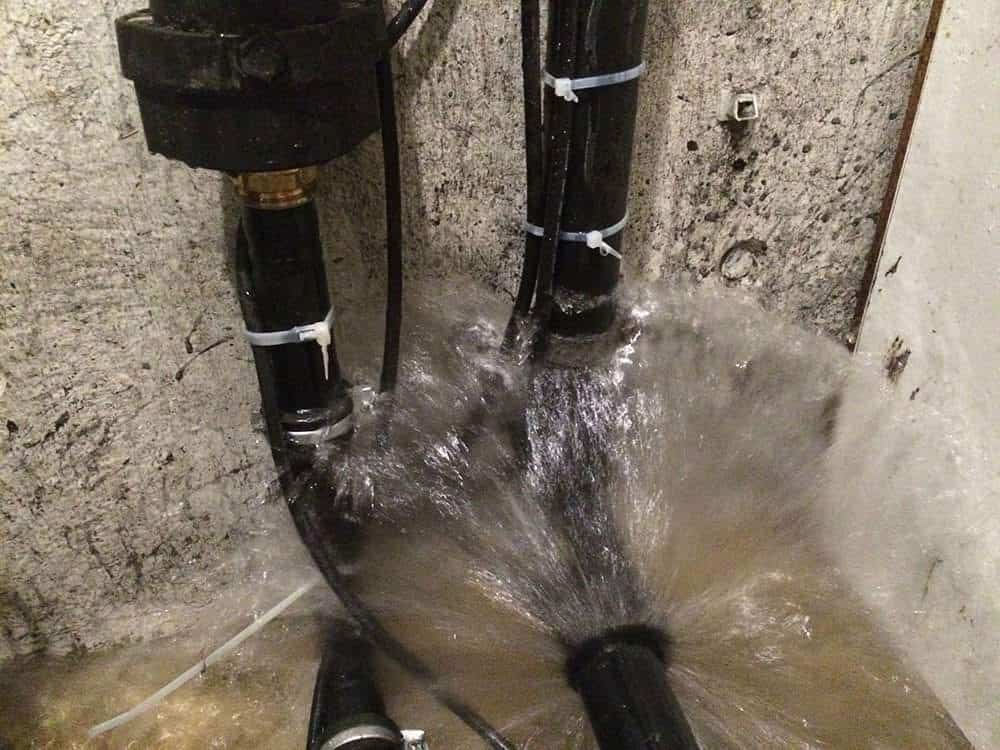The photograph captures two black plastic pipes mounted on a left-side concrete wall meeting a lighter-colored concrete wall at a corner, in what appears to be a behind-the-scenes or maintenance area, potentially under a sink. Both pipes run vertically along the wall before curving; the trouble originates at the curved section of the right pipe, where water is heavily leaking and splashing with high pressure. The surrounding area is significantly affected, as evidenced by the green-colored flood covering the flat concrete surface at the bottom of the image. The left wall is visibly soaked and stained with water splashes, while the right wall, although slightly lighter in color, shows less obvious signs of wetness. The pipes are secured to the wall and smaller tubes using zip-ties, hinting at an attempt at securing or supporting them. The powerful spray of water indicates either a break in the pipe or a failed connection at the elbow joint, which is the focal crisis point of this photograph.